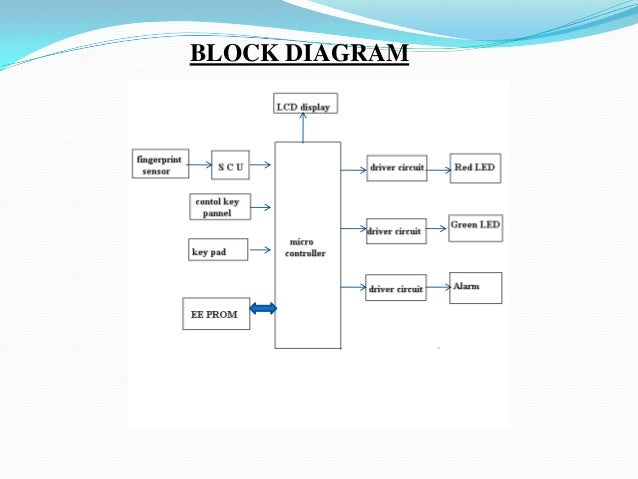The image features a detailed PowerPoint slide titled "BLOCK DIAGRAM," prominently displaying a flowchart. The background is adorned with decorative, wavy blue patterns, adding a visual flair at the top. At the center of the flowchart is a large vertically-oriented rectangle labeled "Microcontroller."

Above the microcontroller, an arrow points upward to a small rectangle that reads "LCD Display." To the left of the microcontroller, two sets of components feed into it. The upper-left section starts with a rectangle labeled "Fingerprint Sensor," which is connected to another rectangle labeled "SCU," and then feeds into the microcontroller. Below this, another row begins with a rectangle labeled "Control Key Panel," followed by a "Keypad" rectangle, both pointing right to the microcontroller. Further down on the left side, a rectangle labeled "EEPROM" connects to the microcontroller with a bi-directional blue arrow.

On the right side, three rows feature rectangles all labeled "Driver Circuit," each connected to an individual element in the second column: a "Red LED," a "Green LED," and an "Alarm," respectively. Arrows flow from the microcontroller to these driver circuits, indicating the direction of data or command flow.

This meticulous layout illustrates various interconnected components and signal pathways, culminating in a well-defined electronic system schematic.